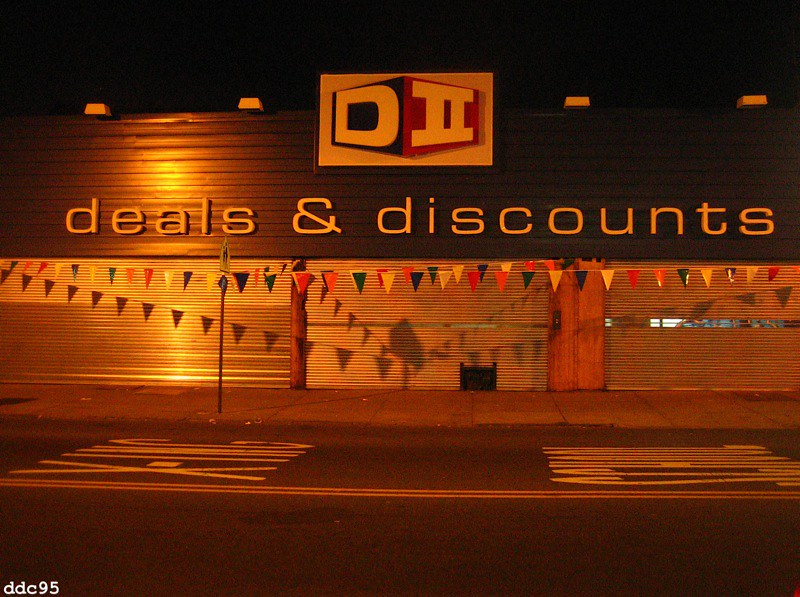The photograph captures a nighttime scene of a storefront. The top portion of the image is enveloped in darkness, gradually revealing the store as you move downward. Dominating the visual is a large, rectangular sign mounted atop the roof. The sign features a white, capital letter "D" on a horizontal rectangle and a Roman numeral "II" on a red background, both prominently displayed.

Beneath this commanding signage, the facade of the store showcases the text "Deals and Discounts" spanning across. The storefront appears newly inaugurated, as evidenced by the festive triangle pennant flags draped around the building's frontage.

Three metal corrugated doors, which resemble garage doors, define the entrance. A wastebasket is visible nearby. The road in front of the store includes a pedestrian crossing and a central dividing line. Finally, at the bottom left-hand corner of the image, the text "DDC 95" is noted, adding a subtle detail to this nocturnal capture.